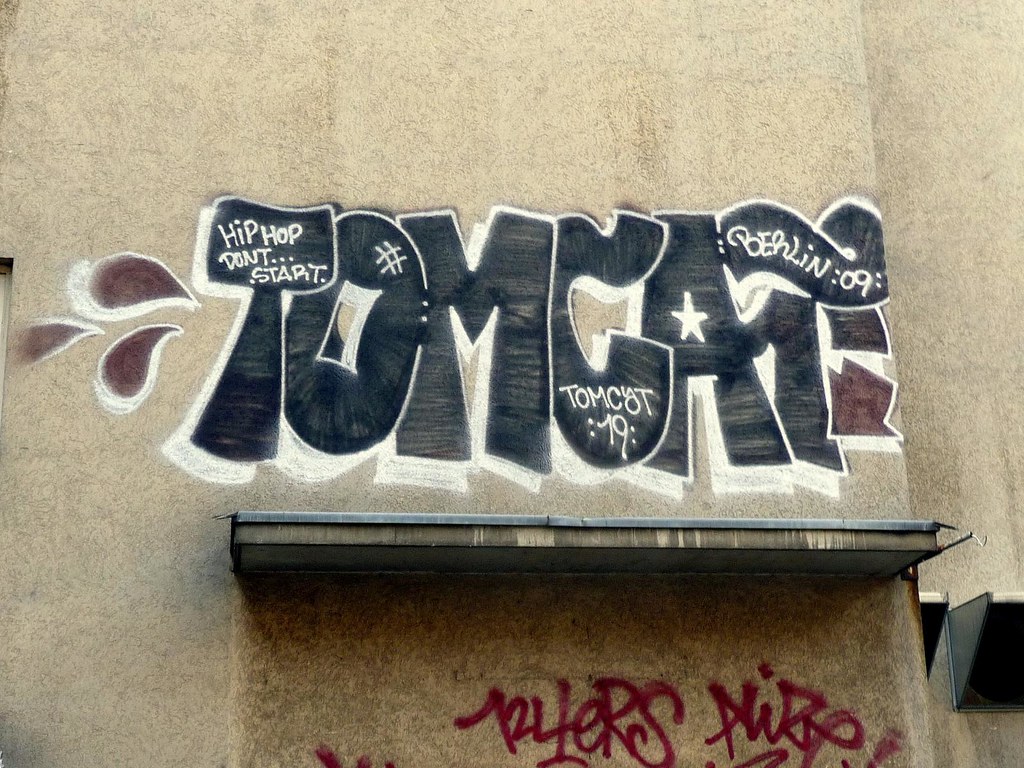The image depicts a graffitied beige or brownish-gray wall under an awning, potentially part of an old or abandoned building. Dominating the scene is a large, cartoony graffiti piece in black letters with white accents spelling "T-O-M-C-A." Within these letters are additional messages and symbols: "hip hop don't period period period start" inside the "T," a pound sign or hashtag inside the "O," "Tomcat 79" inside the "C," a white star inside the "A," and "Berlin-09" inscribed in white on the final "T." Below the main graffiti and beneath the awning, there's a door boarded up and covered in indistinguishable red graffiti. To the left of the black graffiti, there are red teardrops, while on the right side, there are red arrows pointing downward. The overall effect is a vibrant, layered piece of urban art that suggests a playful yet cryptic message.